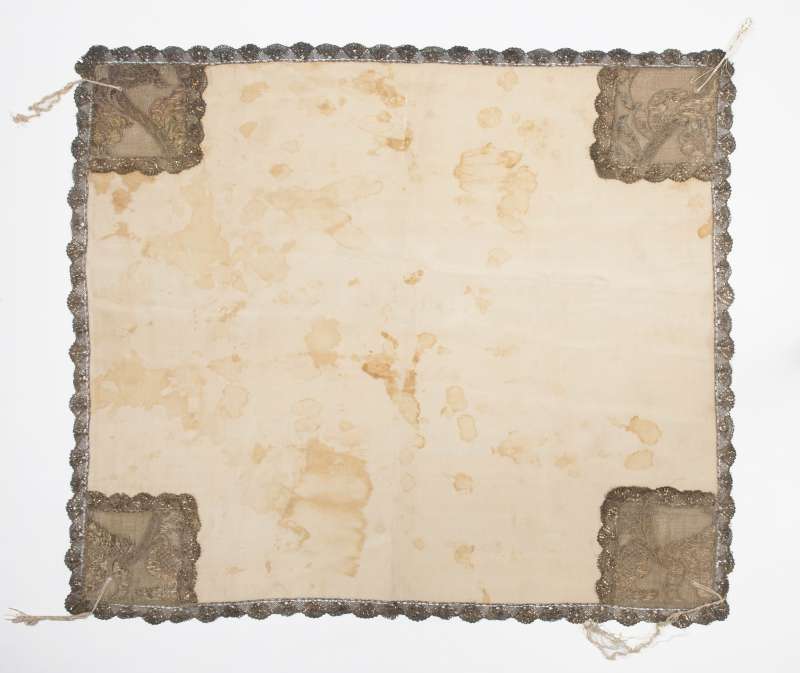The image depicts an antiquated, square piece of fabric or leather, reminiscent of a placemat or perhaps an old stamp. The central area is a tan or dirty beige color, marred with coffee stains and showing signs of aging. The fabric appears to have been cut with zigzag scissors, giving the edges a jagged look. Surrounding the main square are decorative, wavy lacy borders that add a textural contrast. Each corner of the main square features a small brown cutout square, also with zigzag edges, hinting at a once methodical design now slightly frayed and unraveling with loose threads. On the upper right side, a needle is discreetly sticking out, further emphasizing its worn and possibly unfinished state.